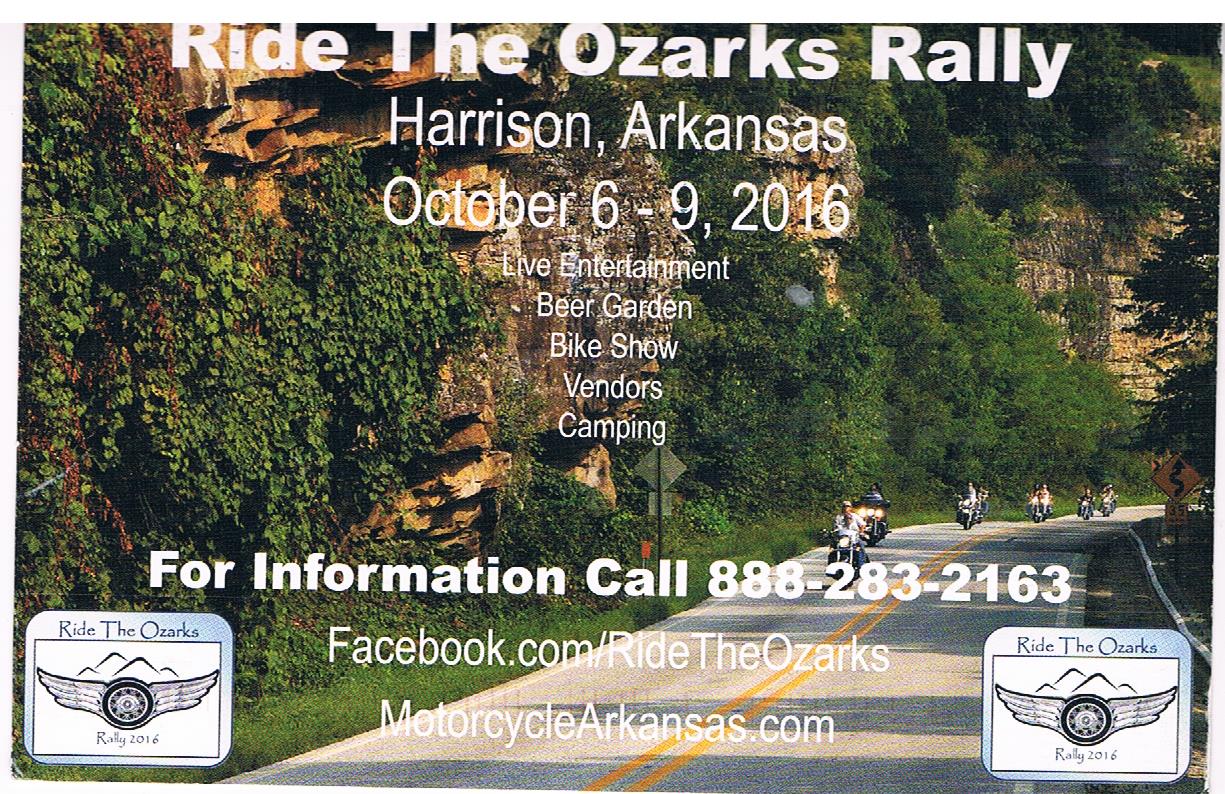The vibrant photograph captures an exhilarating scene from the "Ride the Ozarks Rally," held in Harrison, Arkansas, from October 6 to 9, 2016. Central to the image, six or seven motorcycles roar down a two-lane road marked by a double yellow line, framed by lush green trees and a rocky, ivy-clad incline on the left that forms a natural wall. 

In the bottom corners, the rally's emblem—a tire with wings—appears twice, accompanied by the text "Ride the Ozarks Rally 2016." Bold white text overlays at the top details the main event: "Ride the Ozarks Rally," followed by "Harrison, Arkansas, October 6 to 9, 2016," and highlights the exciting features like "Live Entertainment, Beer Garden, Bike Show, Vendors, Camping." 

Further information is provided at the bottom with the contact number 888-283-2163, along with the website "Facebook.com/RideTheOzarks." The combination of rich natural scenery and dynamic movement of motorcycles perfectly encapsulates the thrill and community spirit of the rally.